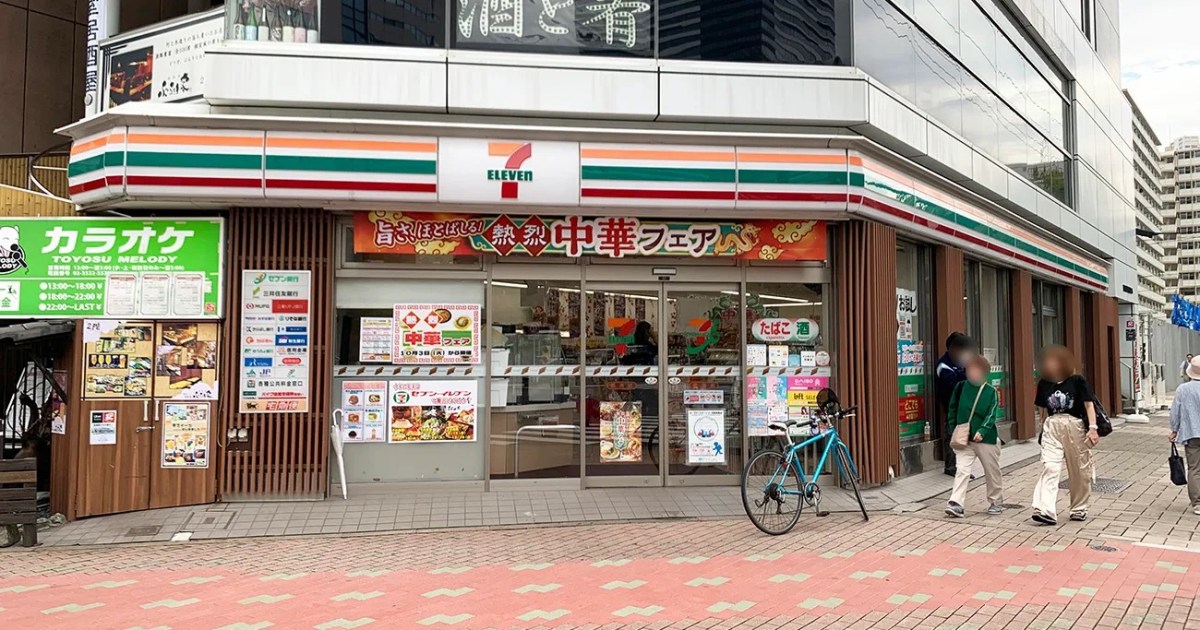The image captures the front of a 7-Eleven store located in an Asian country, possibly Japan, based on the characteristics of the signage and architectural style. The iconic 7-Eleven logo in its familiar yellow, green, and red colors is prominently displayed. Surrounding the logo, there are multiple signs with Asian writing, likely detailing various food products and services offered by the store. A menu board can be seen to the left of the entrance, featuring different food items.

In front of the store stands a light blue bicycle, parked alongside the entrance. A group of three people with blurred faces is visible near the building, ensuring their privacy. One individual, dressed in black clothing, leans against the wall. Another person, wearing a green shirt, beige pants, blue sneakers, and carrying a beige purse, stands nearby. The third individual, also in beige pants but with a black shirt and black shoes, has shoulder-length hair similar to the person in green.

The street in front of the 7-Eleven features a distinctive brick road with light pink bricks. The walkway within the brick road has a unique pattern consisting of salmon-colored bricks with yellow diamond designs. A small section of a wooden bench is visible on the left side of the image. Additionally, the presence of cobblestone with a red line and beige squares adds to the intricate and traditional appearance of the surrounding area. It is daytime, and the scene is bustling with life as people walk by the store.